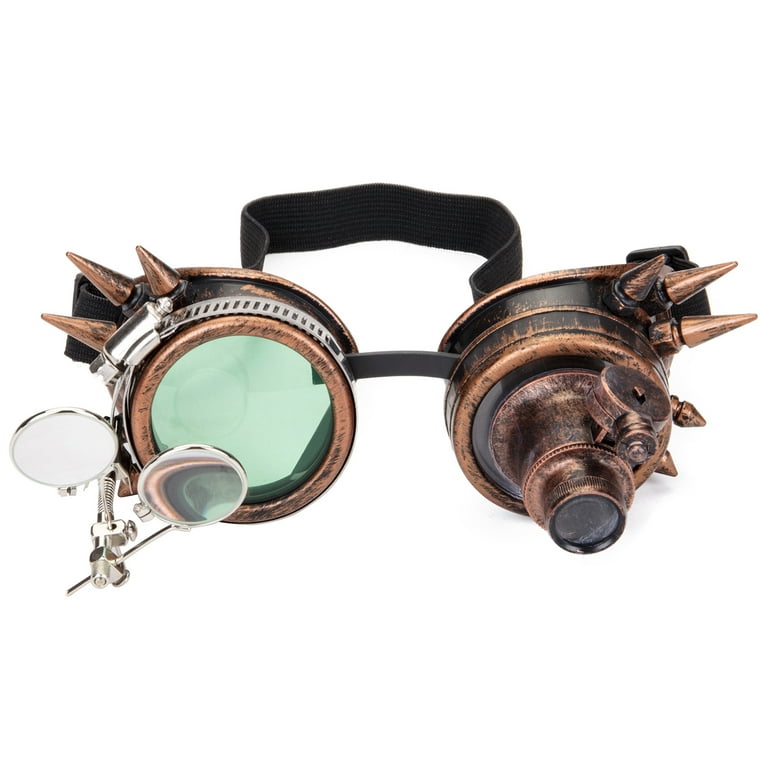The image features a pair of steampunk-styled goggles set against a plain white background. The goggles are crafted from a brass or copper-like metal and are designed with intricate details that evoke an old-fashioned aesthetic. A black strap runs across the back for securing the goggles to the head. The left side of the goggles showcases a clear round lens with two smaller, foldable magnifying lenses that can be rotated in front for enhanced viewing. This lens also includes a clamp and a small spring mechanism, adding to its elaborate design. The right side features a solid metal lens cap, decorated with bronze spikes, giving it a monocle-like appearance. Both lenses are adorned with three decorative spikes on their top edges, reinforcing the steampunk theme. The functional and ornamental elements blend harmoniously, making these goggles a unique and eye-catching piece of craftsmanship.